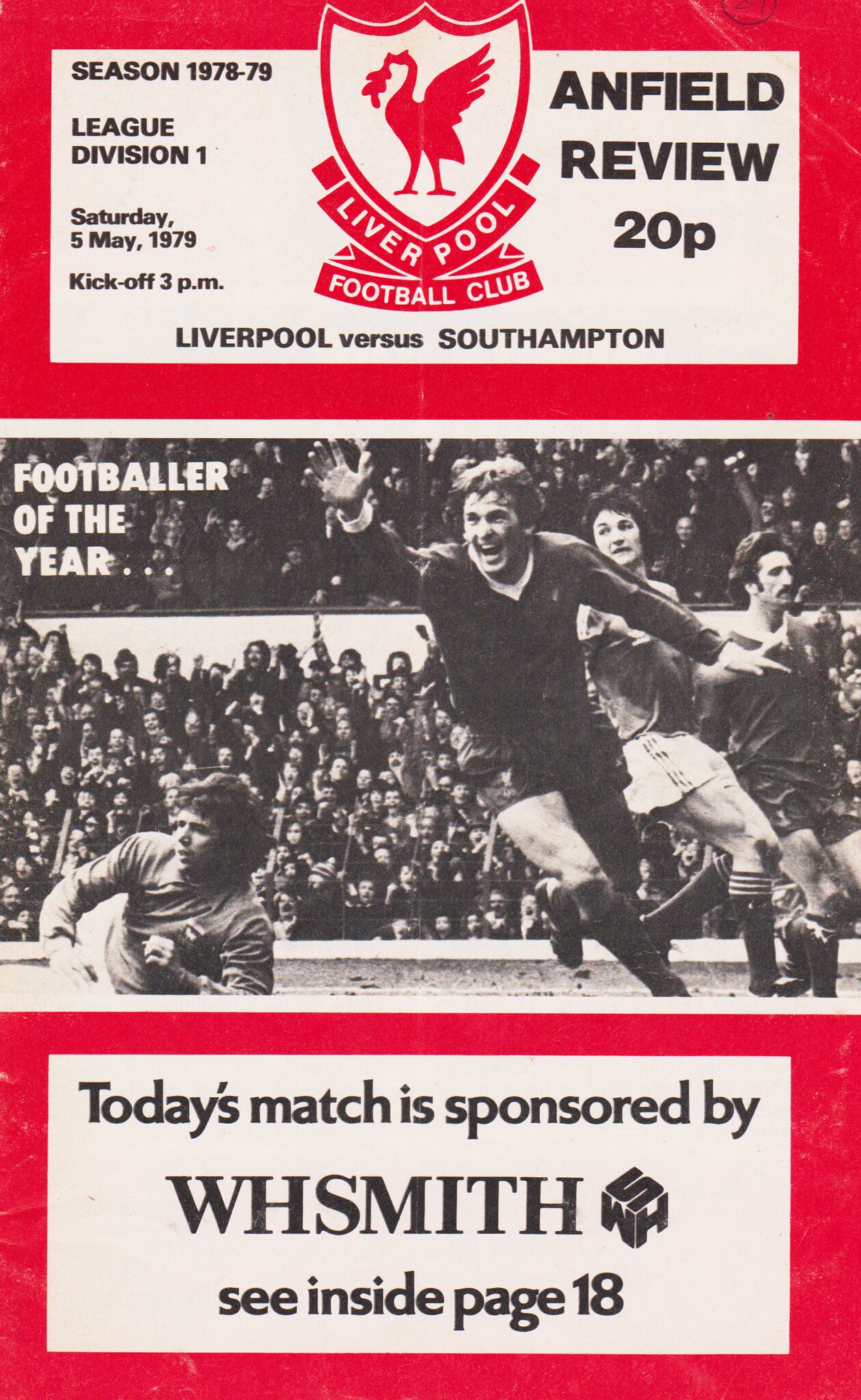This image is a vertical rectangular program from a soccer match, divided into three horizontal sections. The top section features a red border with a white rectangle inside it, containing the Liverpool Football Club logo, which depicts a red and white bird holding an olive branch inside a white shield with a red outline. To the right of the logo, the text reads "Anfield Review 20P" in black, and to the left, it states “Season 1978-79, League Division One, Saturday, 5 May 1979, Kickoff 3 p.m.” Below that, in black text, it says "Liverpool versus Southampton."

In the middle section is a black and white photograph capturing the excitement of a football match. A player is seen celebrating while three other players are visible on the field, one of whom has fallen. In the background, the stands are packed with spectators. The top left corner of the photograph is marked by the text "Footballer of the Year" in white.

The bottom section mirrors the top with its red border and white rectangle enclosing black text that reads, "Today's match is sponsored by WH Smith. See inside page 18."